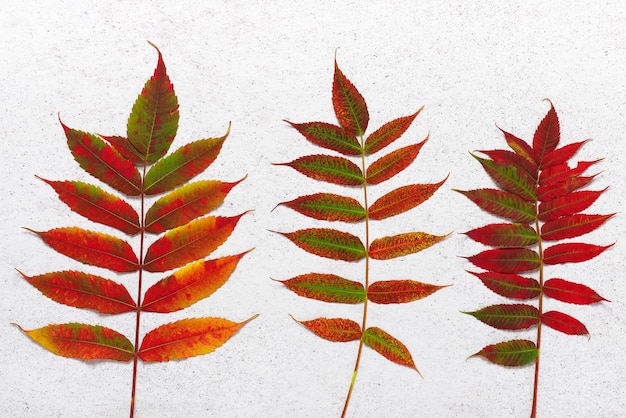The image showcases three meticulously arranged leaf stems, each distinct yet sharing a similar structure and coloring. Positioned side by side with equal spacing on a speckled gray or white background, the stems highlight a harmonious blend of natural hues—incorporating yellows, greens, reds, and variations of pink. The stem on the left holds twelve leaves, the middle stem bears thirteen, and the right stem features eighteen leaves, displaying a progression in the number of leaves from left to right. Each stem bursts forth with leaves that reveal intricate vein patterns in shades of green and red. Additionally, the right stem exhibits a unique coloration pattern where leaves on the right are predominantly red, while those on the left are more green. The detailed shading and meticulous placement of the leaves suggest this is either an artist's creation or a carefully crafted digital image, emphasizing the subtle variations and beauty of each leaf.